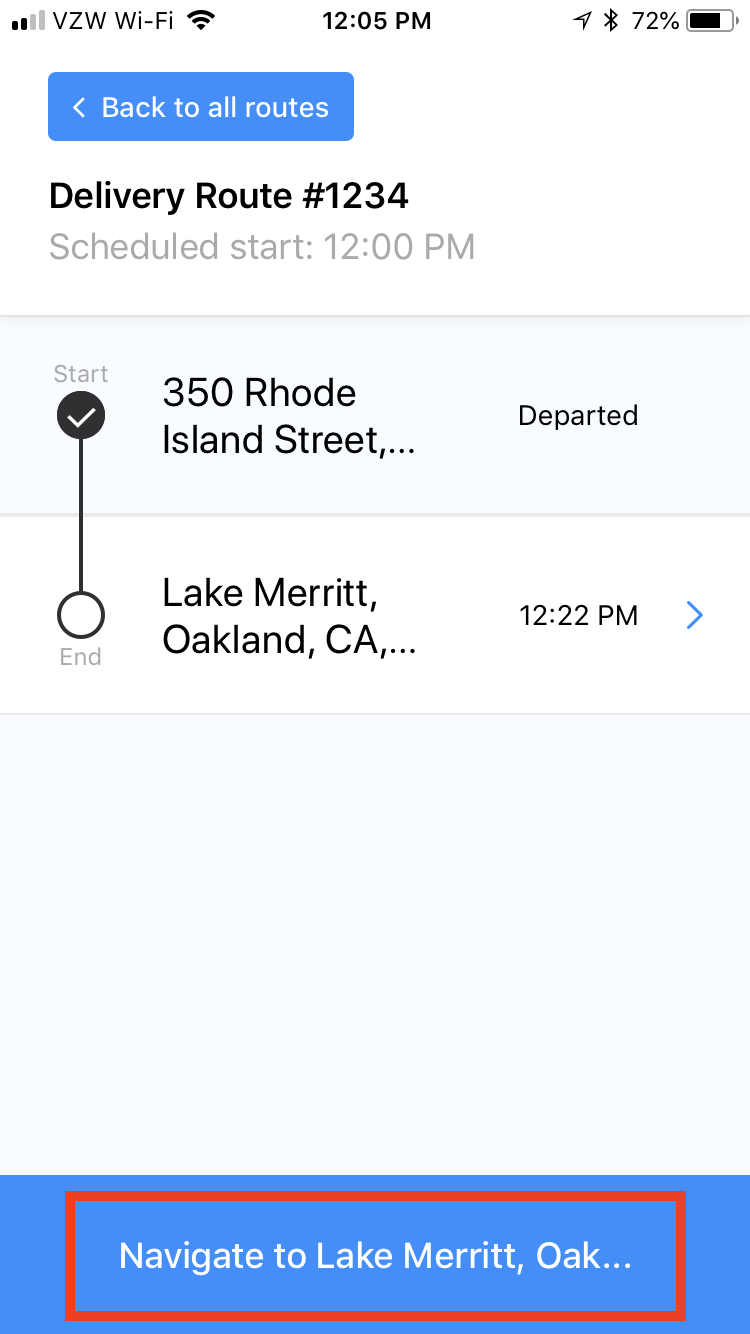At 12:05 p.m., the device displays full bars of Verizon Wi-Fi service with a 72% battery life and a Bluetooth connection. The main screen shows a delivery route interface with a blue button labeled "Back to All Routes." Delivery Route #1234 is scheduled to start at 12:00 p.m. and is marked with a check mark. 

The delivery has departed from 350 Rhode Island Street and is on its way to Lake Merritt, Oakland, CA, as noted at 12:22 p.m. in a white circle beside the location. At the bottom of the screen, there's a red boxed area with white text and a blue button containing a downward-pointing arrow for navigation to Lake Merritt, Oakland.